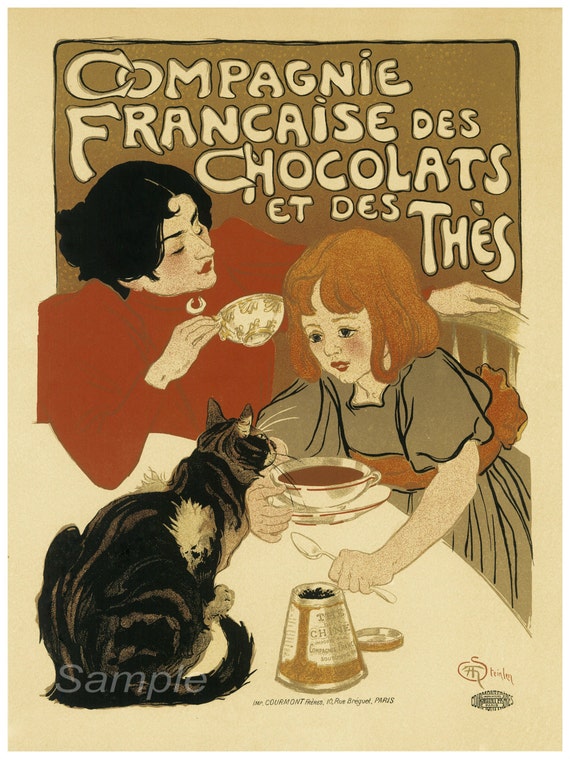The poster, drawing from an old-fashioned style reminiscent of the early 1900s, depicts a scene featuring a dark-haired woman with red lips, dressed in a red blouse with white details at the top, holding a white and beige teacup. Sitting beside her, in a beige chair, is a red-headed girl with shoulder-length hair, clad in a grayish-green dress with a red sash. The girl has a spoon in her left hand and a large cup and saucer resting on the table, containing a brown liquid. A black and white cat with "Sample" written in gray on its tail perches on the table, beside a brown and beige container with its lid off. The whole scene is framed by a beige border, with a smaller black outline inside. At the top of the poster, in tan uppercase letters, the French phrase "Compagnie Française de Chocolat et des Fées" is written. The artist's signature appears at the bottom right corner of the poster.